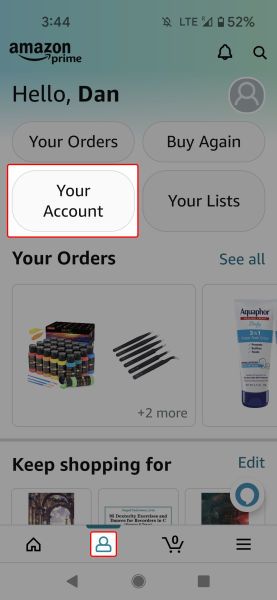This is a detailed screenshot of the Amazon app interface. At the top, it displays the current time, "3:44," and features the "Amazon Prime" logo next to an avatar icon labeled "Heldan." Below this, there's a button labeled "Your Orders," which is highlighted and positioned to the right. Beneath "Your Orders," there's another button labeled "Your Account," presented in white and surrounded by a red box. To the right of "Your Account" is a button labeled "Your Lists."

Directly underneath "Your Account," the "Your Orders" section is suggested again. Adjacent to this, a section with colorful paints and markers in a box is shown, which includes a notation of "2+ more." To the right of this, an image of an "Aquaphor lotion bottle" is displayed. Following these images, the phrase "Keep Shopping Forward" is displayed, leading into three more product images. 

To the right of these images is a blue and white action button. At the bottom of the screen, a navigation bar features several icons: a "Home" button, a "Person" button (white with a red outline), and a "Shopping Cart" button with three lines. Notably, all elements on the screen, except for the two white buttons, have a grey overlay.